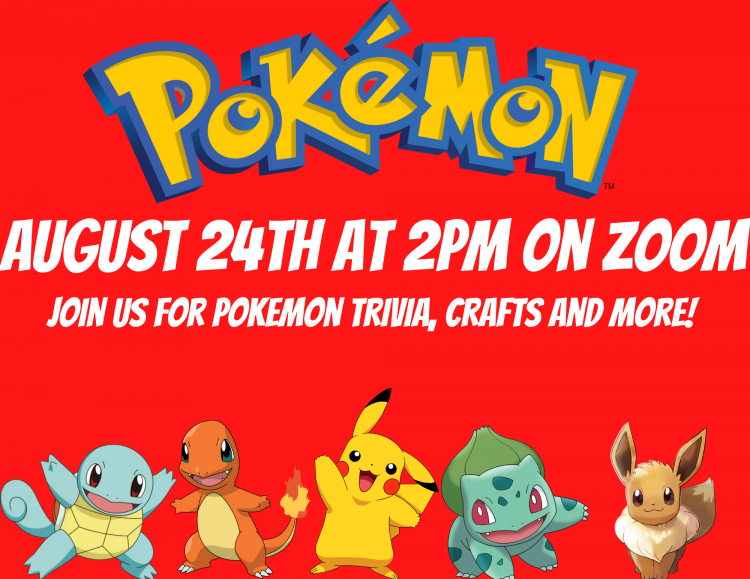This vibrant Pokémon poster features a striking red background. At the top, bold "Pokémon" text is prominently displayed with a blue outline, yellow interior, and highlighted edges to give a 3D effect. The iconic accent mark over the "é" and a small "TM" located at the end of the word are also visible.

Below the title, in all-caps white lettering, is the event information: "AUGUST 24TH AT 2 P.M. ON ZOOM." Beneath that, in slightly smaller but still all-caps white text, reads: "JOIN US FOR POKEMON TRIVIA, CRAFTS, AND MORE!"

Occupying the lower section of the poster are five well-known Pokémon characters, each distinctively illustrated. From left to right:

1. **Squirtle**: The blue, turtle-like Pokémon with his light yellow tummy stands with raised arms, exuding a playful energy.
2. **Charmander**: This small, orange dinosaur-like Pokémon features a fiery tip on his tail and stands with arms outstretched.
3. **Pikachu**: Centrally positioned, Pikachu, the yellow electric Pokémon, brings enthusiasm with his right arm up, left arm down, and asymmetrical ears (right ear up, left ear down). His red cheeks and open mouth reveal his cheerful spirit.
4. **Bulbasaur**: The green and blue Pokémon, with a bulb on his back and darker blue-green spots, is smiling broadly. His right front arm is lowered while his left stretches forward.
5. **Eevee**: At the far right, the brown, fox-like Pokémon stands with both front legs together, fluffy white chest fur, ears perked up, and a visible bushy tail.

Notably, all characters but Eevee have open mouths displaying pink interiors. Pikachu, Squirtle, Charmander, and Bulbasaur boast black eyes, while Bulbasaur's eyes are a dark red, and Eevee’s are brown.